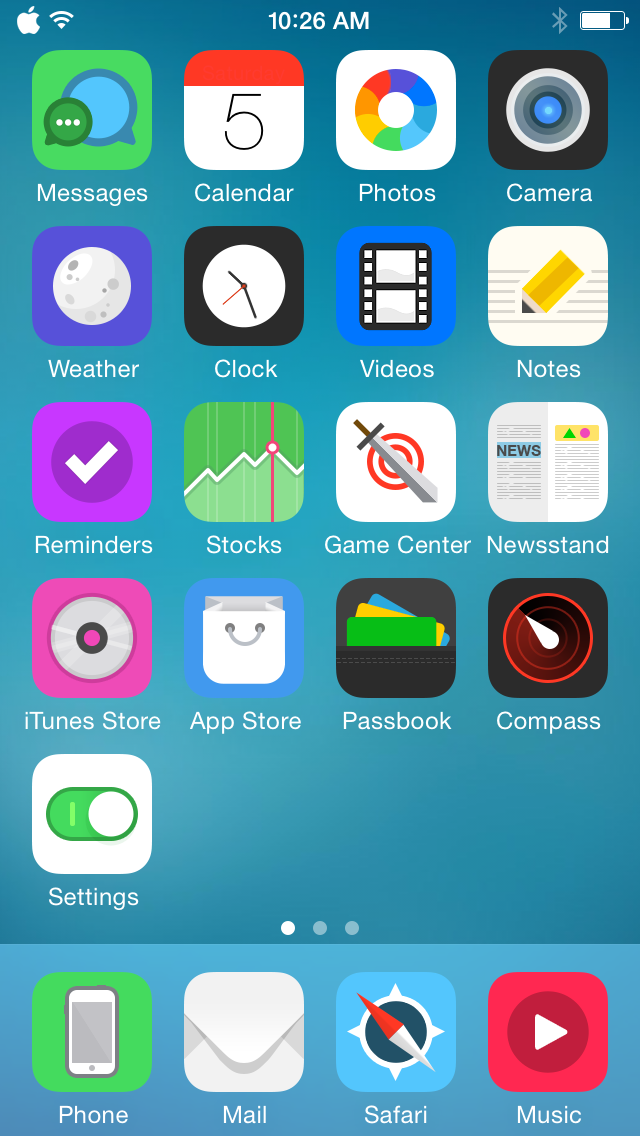This screenshot captures the home screen of a smartphone, specifically the first page of app icons and wallpaper. Displayed at the top of the screen is the time, which reads 10:26 AM. Below the time, the screen is divided into five rows of app icons. The top row features the following applications: Messages, Calendar, Photos, and Camera. The second row displays icons for Weather, Clock, Videos, and Notes. In the third row, you can see Reminders, Stocks, Game Center, and Newsstand. The fourth row contains the iTunes Store, App Store, Passbook, and Compass. The fifth and final row appears to be a single widget or settings icon, which is a white square with a green toggle button in the center. The overall layout and application arrangement provide a clear and organized view of essential apps for easy access.